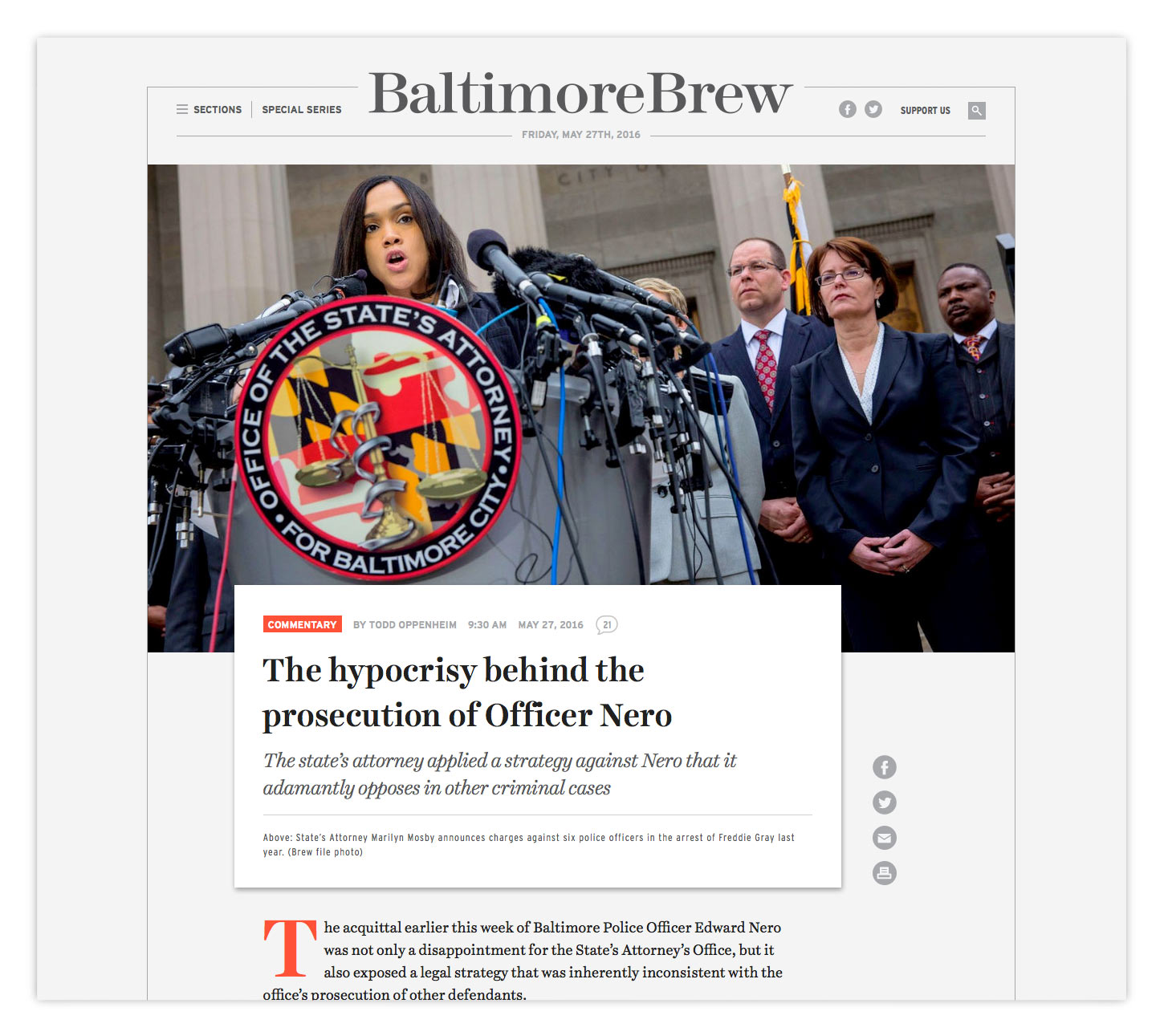Sure, here is a cleaned-up and detailed caption:

---

**Desktop Screenshot of a News Article from "Baltimore Brew"**

The screenshot captures a desktop view of a news article from "Baltimore Brew," dated Friday, May 27, 2016. The top middle of the screen prominently displays the publication name in a gray background. To the left of the title, there are links labeled "Sections" and "Special Series." On the right side, icons for Facebook and Twitter are present, followed by "Support Us" and a magnifying glass icon for search functionality.

Below the header, an image shows a woman speaking at a podium equipped with multiple microphones. The podium displays the insignia, "Office of the State's Attorney for Baltimore City." Four individuals stand behind her, and the setting appears to be outside a significant government building, likely near the mayor’s office or a courthouse.

Further down, the article's details reveal a commentary by Todd Oppenheim, posted at 9:30 a.m. on May 27, 2016, with 21 comments indicated by a thought balloon logo. The article is titled "The Hypocrisy Behind the Prosecution of Officer Nero." In a smaller font, it notes, "The state's attorney applied a strategy against Nero that it adamantly opposes in other criminal cases." The article describes how the acquittal of Baltimore police officer Edward Nero earlier in the week disappointed the state’s attorney's office and highlighted an inconsistent legal strategy compared to other prosecutions.